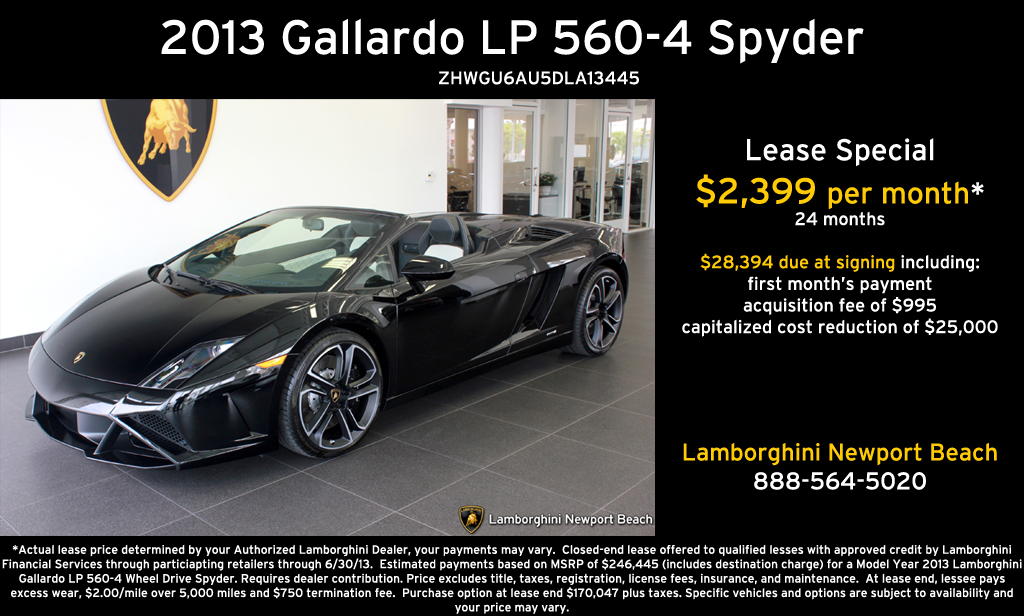This advertisement features a striking image of a gleaming black 2013 Lamborghini Gallardo LP560-4 Spyder in a showroom. The convertible sports car, showcased against a white wall adorned with what appears to be the Lamborghini logo, stands out on glossy black tiles. Glass doors and dividers in the rear hint at office spaces. The bold text at the top details the model and a serial number. Highlighting the lease special, it offers the car at $2,399 per month for 24 months, with $28,394 due at signing. This amount includes the first month's payment, an acquisition fee of $995, and a capitalized cost reduction of $25,000. The advertisement, promoting Lamborghini Newport Beach, also features contact information and legal terms at the bottom.